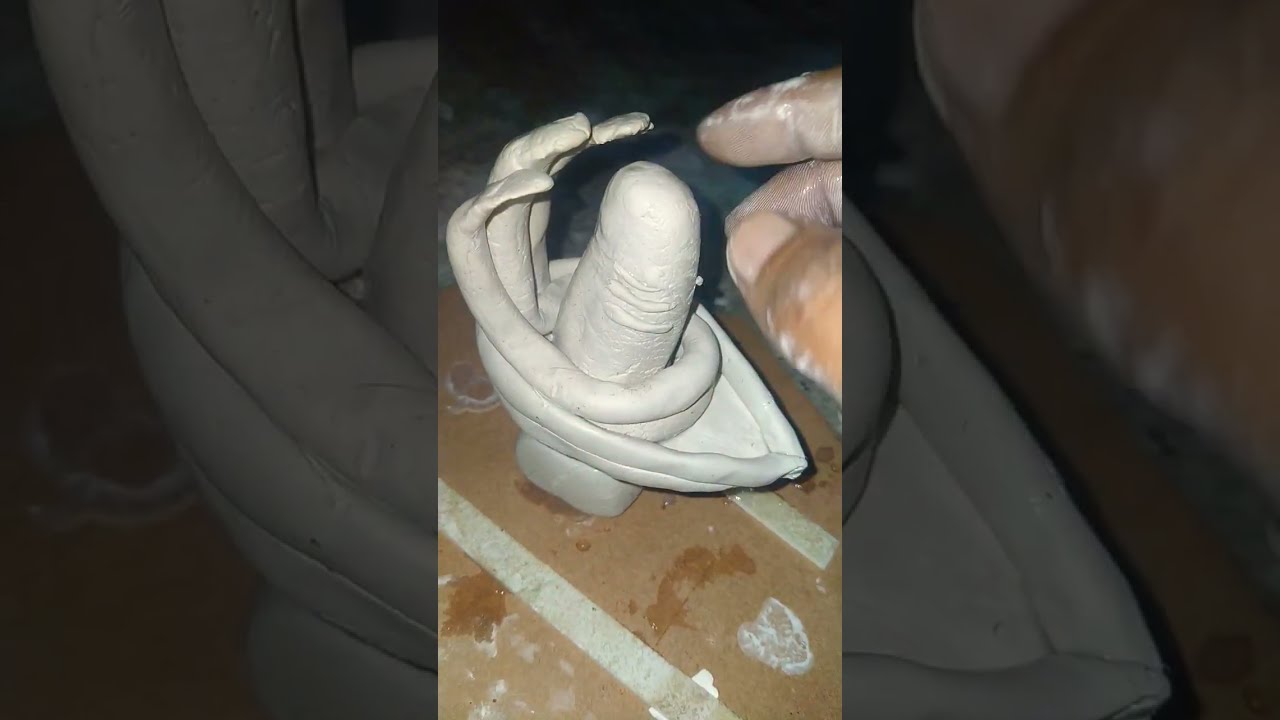The image captures an intriguing clay art project that a dark-skinned person is actively working on. The creation, peculiar and difficult to precisely identify, is an abstract sculpture formed of a grayish-white, possibly bluish gray clay, positioned centrally in the frame. The sculpture somewhat resembles a chair or a toilet seat with a finger protruding from it, surrounded by undulating lines reminiscent of tidal waves or tentacles. The sculptor's hand, smeared with clay, is visible in the upper right corner, indicating they have been molding and shaping the piece. The sculpture sits on a brown wooden board or cardboard, slightly wet and taped, suggestive of recent work in what appears to be an art studio. The backdrop is a textured gray marble surface, adding to the studio ambiance. The image appears to be a screenshot from a video where the artist might be displaying their finished or nearly completed piece.